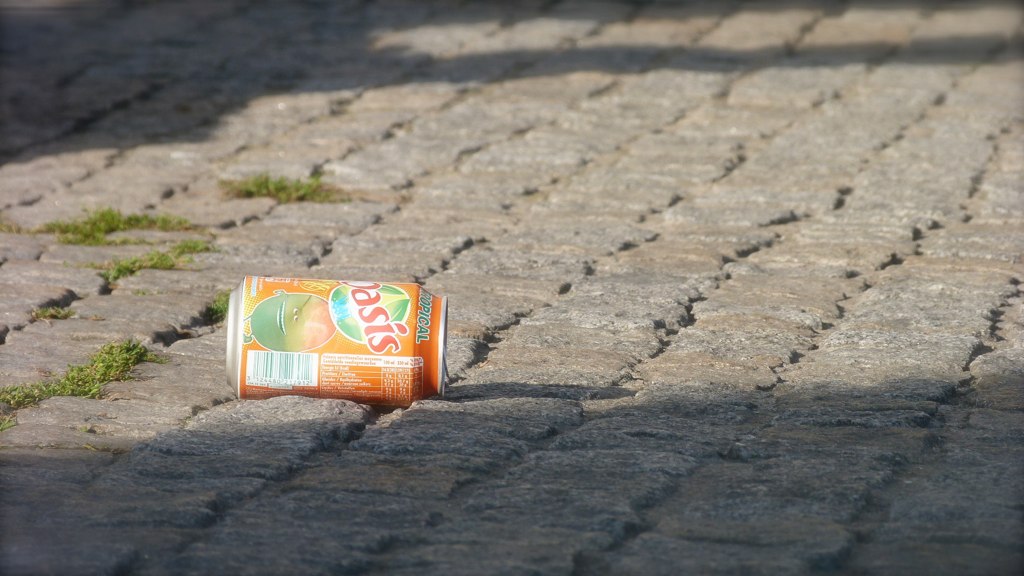This photograph captures a solitary scene of a cobblestone street bathed in sunlight. A bright orange soda can featuring the brand name “Oasis” in red letters is prominently displayed, lying on its side slightly left of center. The can is adorned with the word “Tropical” across the top in green letters and showcases an anthropomorphized fruit resembling an orange with a mouth and small eyes. The detailed can also includes visible nutrition facts and a barcode. The sunlight highlights the can's features, casting its shadow to the right, suggesting the light source is from the left. The cobblestones are clean, with only sparse patches of grass peeking through on the left side, adding a touch of nature to the otherwise stone-paved ground. Surrounding shadows frame the photograph at the top and bottom, creating a contrast with the illuminated central area.